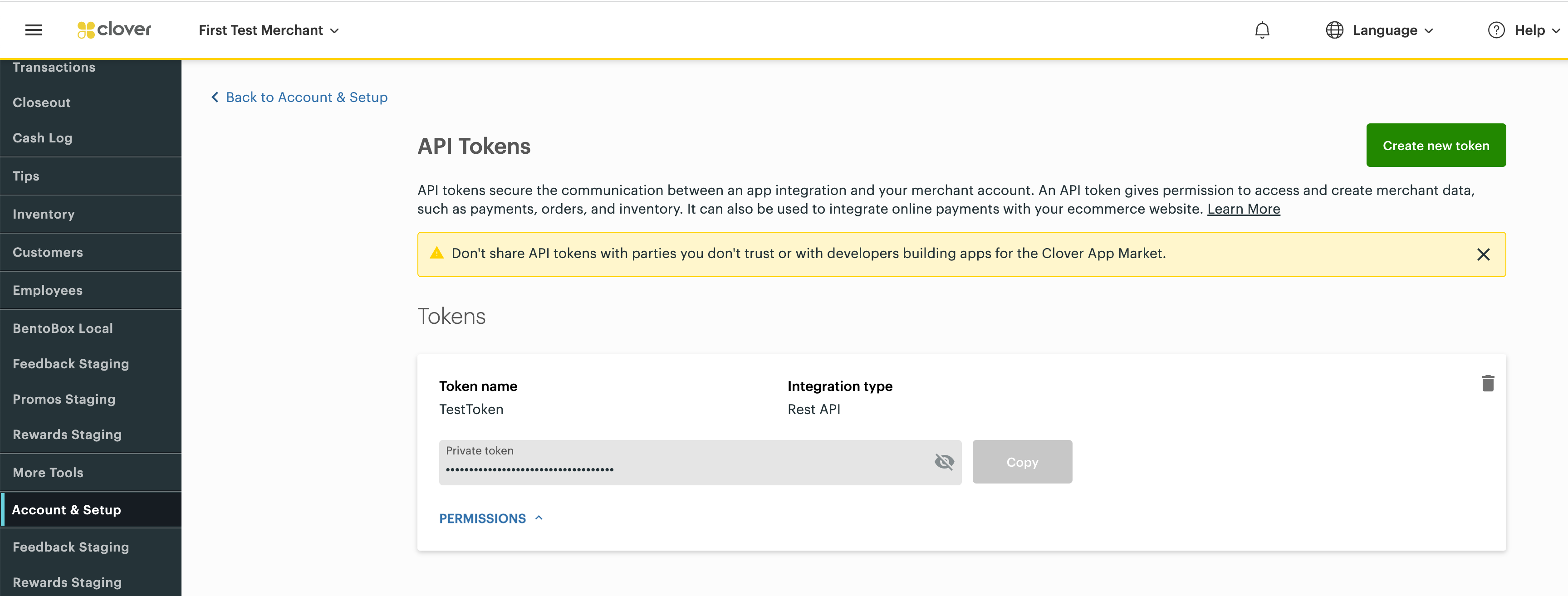The web page features a minimalist design, dominated by a clean white background and sleek black text. At the very top left corner of the page, there is a small square icon. Adjacent to this icon is a yellow "N" followed by the word "Clover" in lowercase letters; next to this, the phrase "First Test Merchant" is displayed. On the top right corner, there is a globe icon labeled "Language" for selecting different languages, followed by a circular icon with a question mark, labeled "Help."

Below this header, a vertical navigation menu is situated along the left-hand side within a black rectangular box, which is wider than it is tall. This menu contains white text and lists various options such as "Closeout," "Cash Log," "Tips," "Inventory," "Customers," "Employees," and "Feedback Staging."

In the main content area, centered prominently, the heading "API Tokens" is visible. Positioned to the right on the same line is a green button labeled "Generate Tokens." There is also another section below, featuring a text box labeled "Tokens," which contains a dropdown menu for further selections or actions.